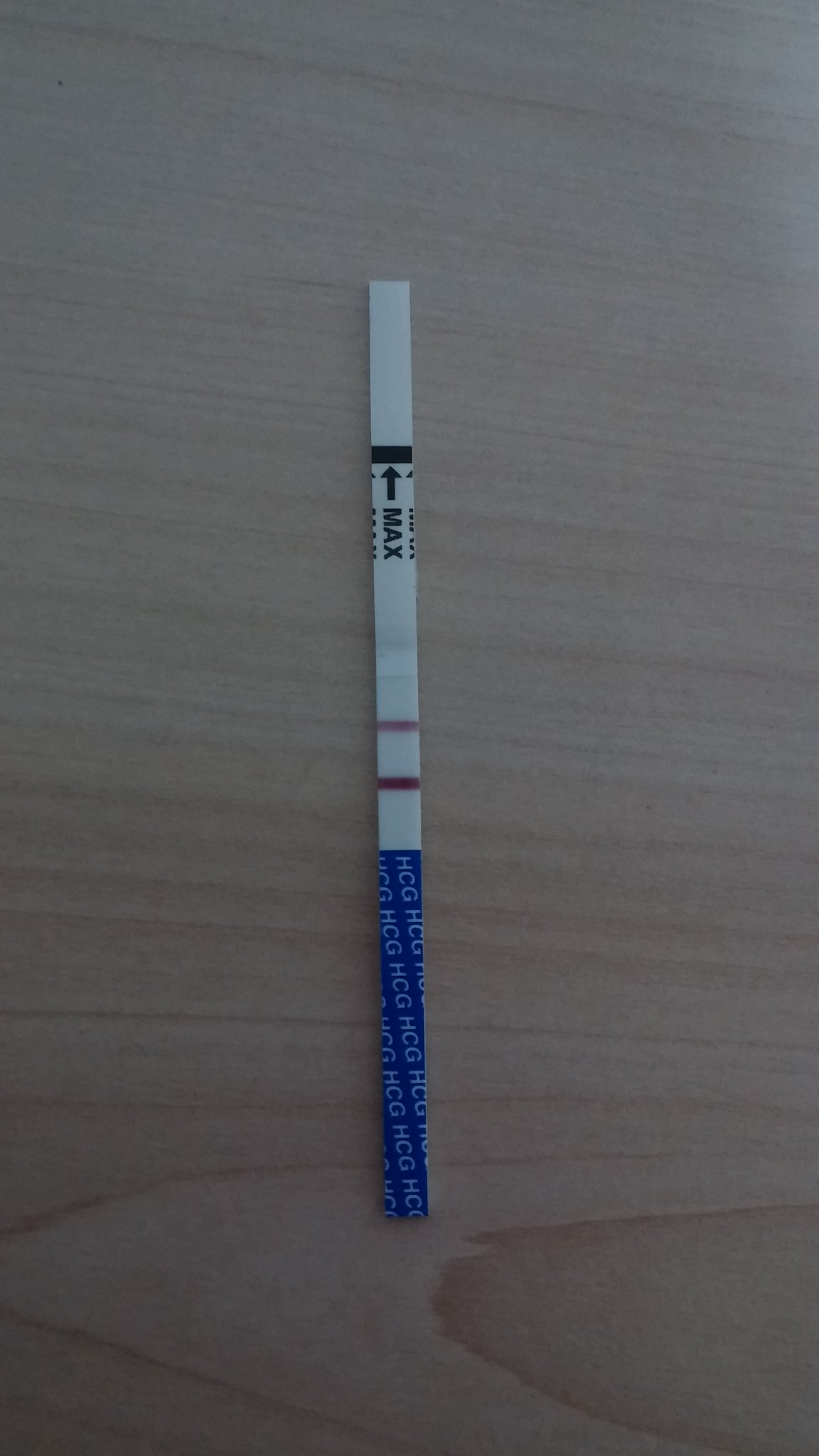This real-life close-up photograph captures a slender testing strip resting on a textured wooden surface characterized by a beige hue with darker brown grain patterns. The strip occupies the centerpiece of the image, drawing attention with its intricate details. 

The upper 60% of the strip is predominantly white. Near the top, a horizontal black line traverses the width of the strip. Adjacent to this line, the word "MAX" is written in all capital letters, oriented sideways, alongside an arrow that points to this black line. The white expanse continues below this marking.

Approximately midway down, a faint brick-red stripe cuts across the strip, reminiscent of the markings on a pregnancy test or a chemical testing strip. This is followed by another white section that extends into a more distinct, darker red band. A small segment of white appears below this red stripe before transitioning into the bottom 40% of the strip, which features a royal blue background.

The blue section is densely patterned with the letters "HCG" printed in white, arranged diagonally and repeatedly, appearing around 12 to 13 times across the entire blue area.

The purpose of the strip is unclear from this image, but the detailed visual description suggests it could be related to testing, possibly in a medical or scientific context.